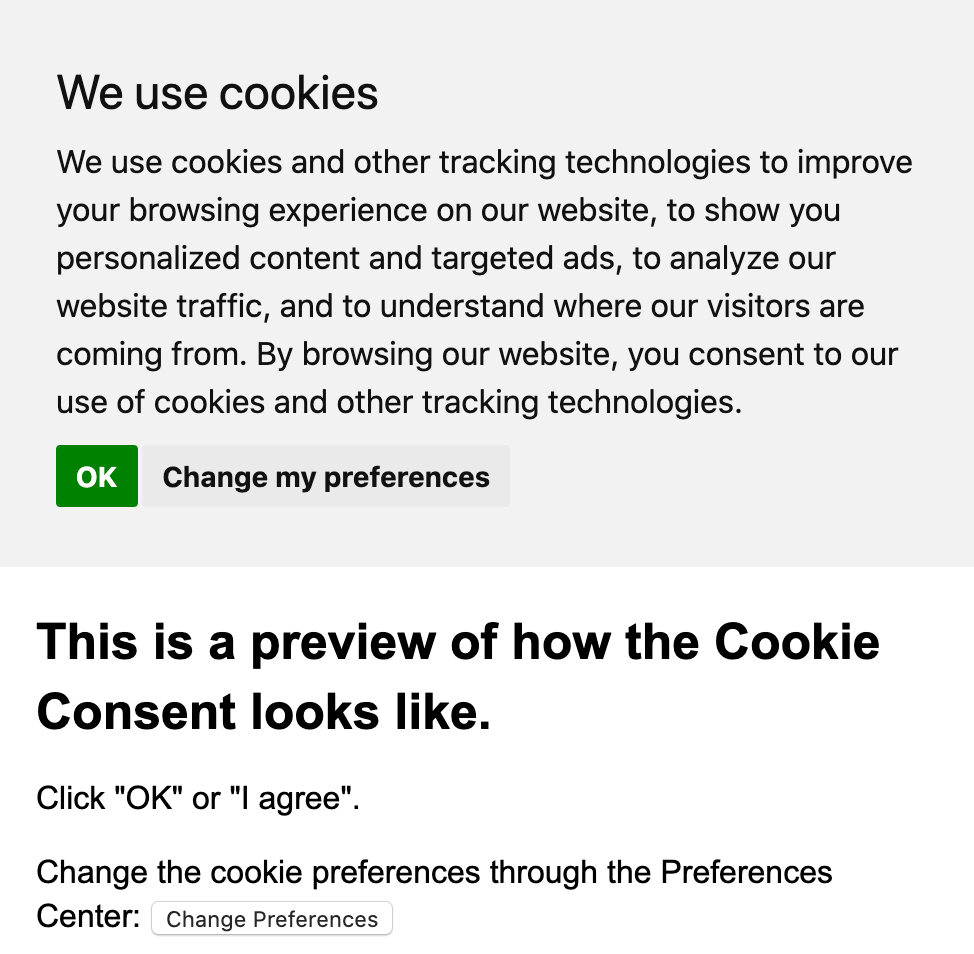This rectangular image displays a vertically-aligned notification about cookie usage. The primary section features a light gray box filled with black text, which reads: "We use cookies and other tracking technologies to improve your browsing experience on our website, to show you personalized content and targeted ads, to analyze our website traffic, and to understand where our visitors are coming from. By browsing our website, you consent to our use of cookies and other tracking technologies." Below this text, there's a green button labeled "Okay," and to its right, there's a link labeled "Change my preferences."

Beneath the gray box, the background shifts to white. In bold print, a message states: "This is a preview of how the cookie consent looks like. Click 'Okay' or 'I agree.' Change the cookie preferences through the preferences center." Below this message, there's another white box outlined in gray that contains the text "Change Preferences." The image is straightforward and functional, primarily aimed at demonstrating the appearance and options of a cookie consent notification.